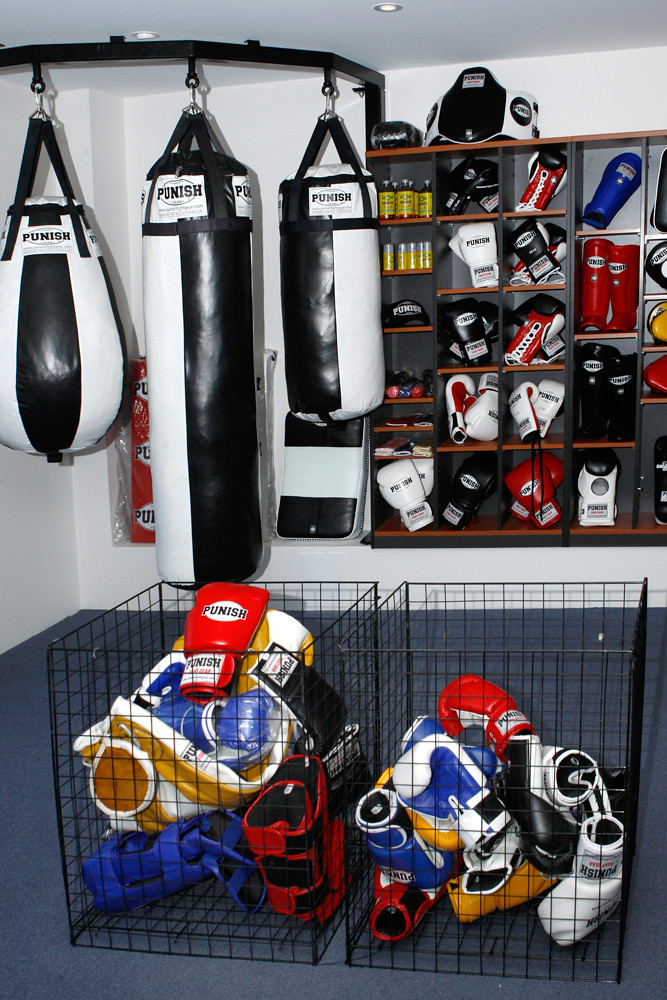This detailed image depicts a well-equipped boxing room with a predominantly white aesthetic, featuring both the walls and ceiling. The ceiling is accented with silver circular light fixtures that provide illumination. In the background, a shelving unit is organized against the wall, displaying a variety of boxing accessories including gloves in multiple colors—black, white, red, yellow, and blue—boots, and possibly bottles for chalk or powder. At the top of this shelving unit, a black and white belt is prominently displayed.

In the middle to left section of the room, suspended from a black metal frame attached to a curved section of the wall, are three punching bags of varying designs and sizes. The central punching bag is a long cylindrical shape, while the one on the left is smaller and tapers from a narrow top to a wider bottom. The right punching bag is also a cylinder but shorter than the central one. All punching bags are predominantly black and white.

In the foreground, there are two wire mesh bins similar to open-top dog cages. The left bin is filled to the brim with an assortment of multi-colored boxing gloves and some protective gear, while the right bin is only half full, housing similar items. The room's floor is blue, contrasting with the otherwise neutral and monochromatic color scheme of the space.